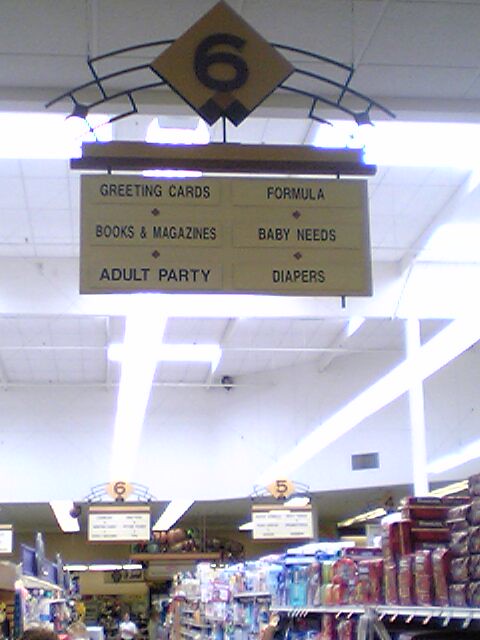A brightly lit grocery store aisle, identified as aisle number six, presents a peculiar mix of products. On one side, shelves are stocked with baby needs, including various diapers, while the opposite side features an assortment of greeting cards, books, magazines, and adult party supplies. The juxtaposition of baby essentials next to adult party items creates an unusual and somewhat disorienting shopping experience. The intense overhead lighting contributes to an almost surreal atmosphere, reminiscent of the eerie 'backrooms' aesthetic.